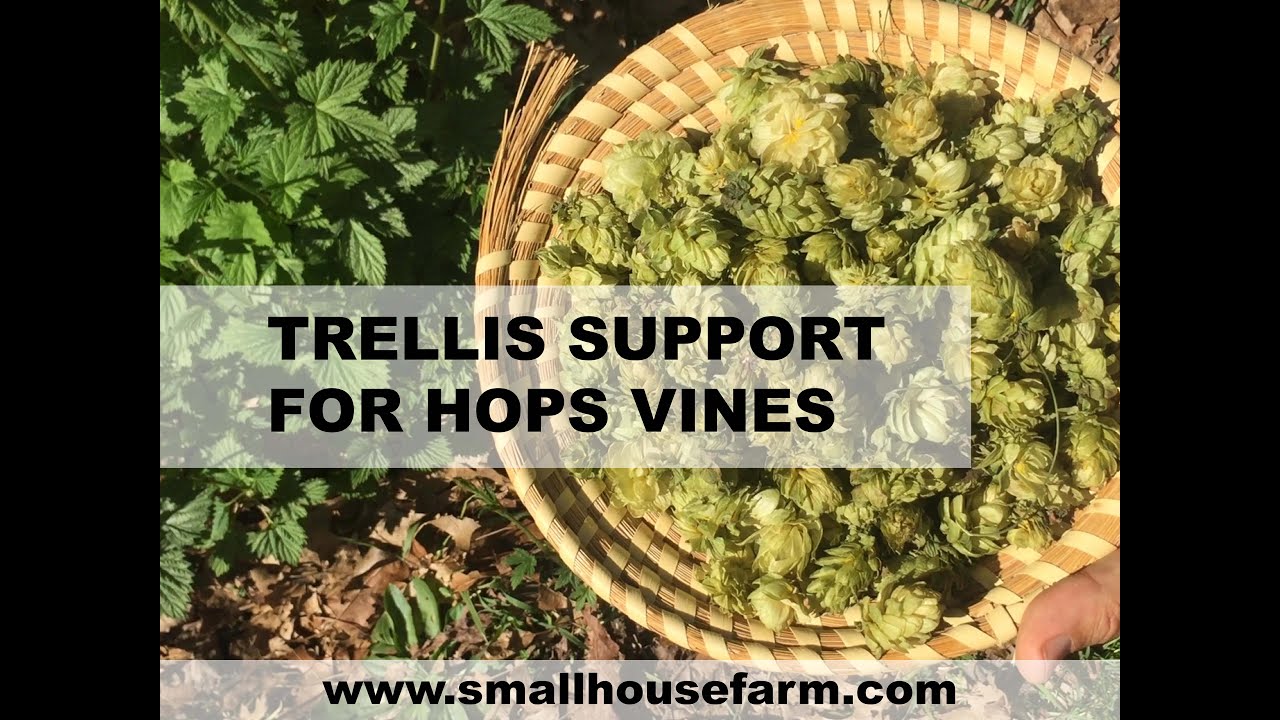The advertisement features a photo taken from above, showcasing a woven, handmade basket with two-tone beige and white strands spiraling in a snail-like pattern. The basket, held by a pair of partially visible hands, contains green, round plant heads resembling Brussels sprouts but with looser leaves, similar to artichokes. Surrounding the basket, the ground is dotted with green plants and patches of dirt. Superimposed in the middle of the image is a transparent text box with black letters stating "Trellis Support for Hops Vines," while a banner at the bottom displays the website "www.smallhousefarm.com."